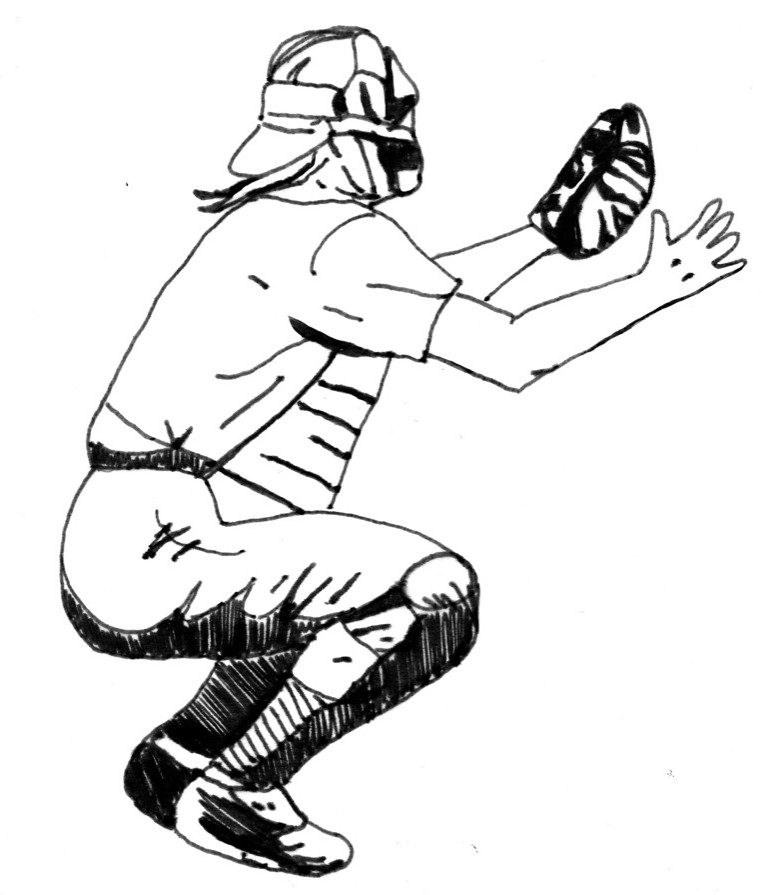This detailed black and white pen and ink illustration depicts a baseball catcher in profile view, squatting down in a typical catcher's stance. The catcher is shown from his right side, with both arms stretched forward as if ready to catch a ball or signal. His left hand dons a catcher's mitt, while his right hand is bare. He is fully equipped with protective gear: a catcher's mask, a short-sleeved shirt, and padding on his chest, held in place by a band around his waist, as well as additional padding on his knees. The catcher appears to be wearing black pants with striping up the back and possibly tall socks. His footwear is some kind of cleat-like shoe. Notable details include a baseball cap worn backwards and long hair streaming out the back. Despite the simplicity of the illustration, the essential features and posture of the catcher are clearly captured.